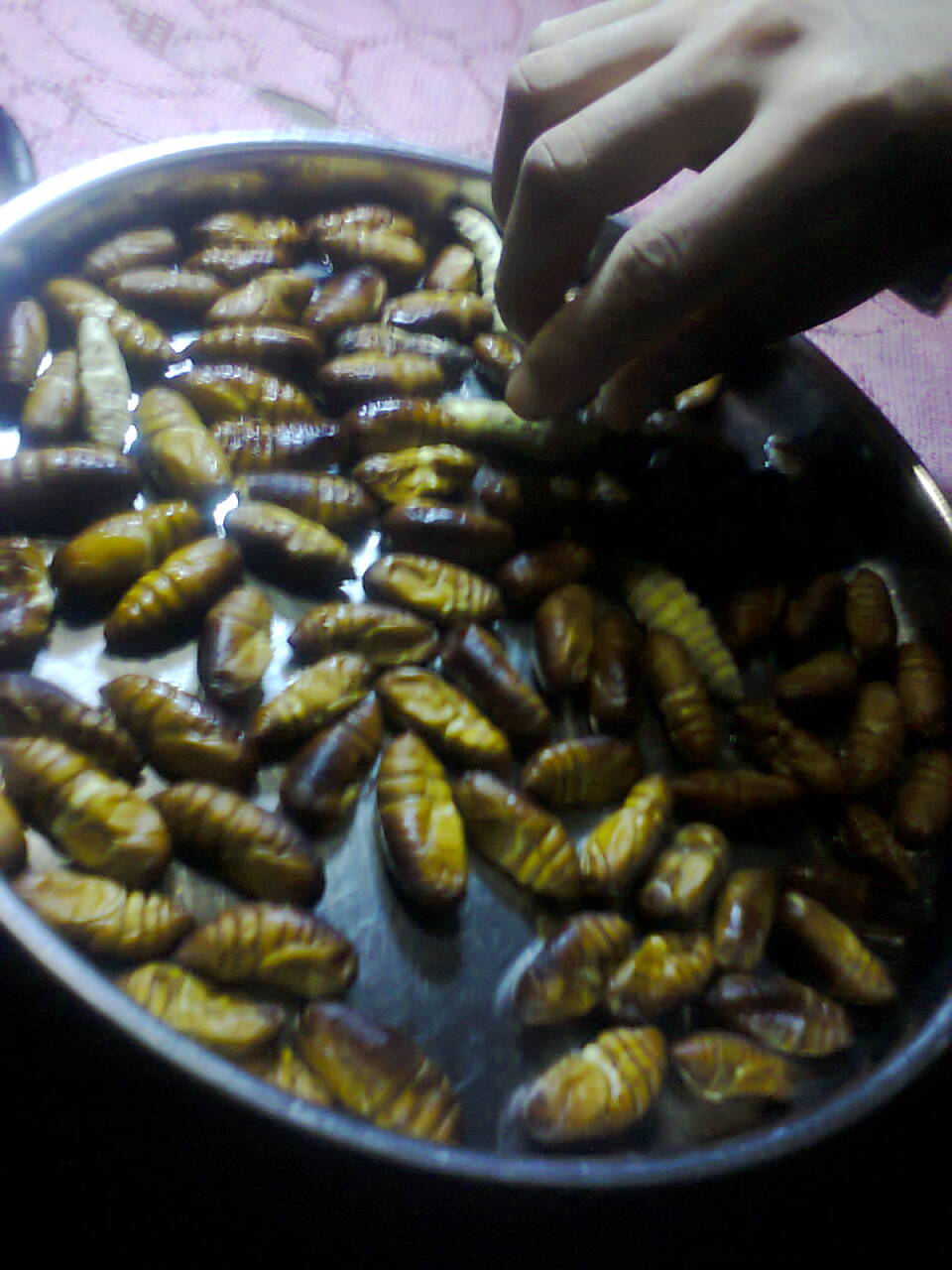The image depicts a close-up of a metallic plate overflowing with toasted brown and yellow insects, possibly grubs or beetles, numbering between 50 and 80. The insects are likely about an inch and a half long, with a shape resembling elongated footballs or small loaves of bread. The scene is set on a marbled tabletop with a pink tablecloth that has a small hole at the top. A brown hand with short nails is reaching into the upper right corner of the frame, poised to pick up one of the bugs, suggesting imminent consumption. The sun casts a reflection on the metal plate, illuminating the darkened, cooked insects.